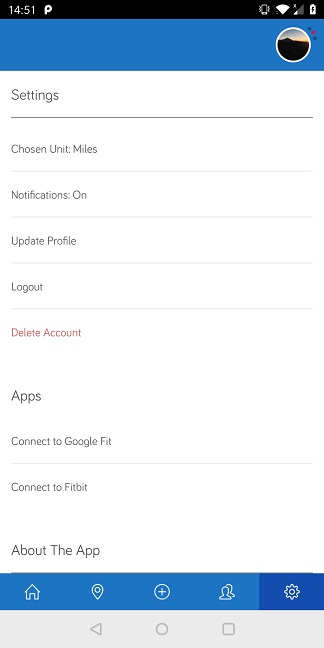**Descriptive Caption:**

This is a detailed screenshot of a smartphone displaying a user interface, predominantly characterized by several colors and sections. At the very top, a black status bar contains the current time and various phone icons. Just below this, a medium blue header spans the width, featuring a sunset-over-mountain profile picture on the right.

The main body of the page has a white background with multiple rows of information categorized under different sections. The first section, "Settings," is in gray text with a horizontal line beneath it. This section includes:
1. Chosen unit: miles
2. Notifications: on
3. Update profile
4. Log out
5. Delete account (in red text)

Following the settings, there is a section for "Apps Information" with two rows:
1. Connect to Google Fit
2. Connect to Fitbit

Subsequently, the "About the App" section appears, however, it does not contain any rows beneath it.

At the bottom, a blue tab features five navigational icons each outlined in white:
1. Home (house icon)
2. Location/Map (balloon-shaped pin with a circle in the middle)
3. Add (plus sign within a circle)
4. People/Accounts (two head-and-shoulder silhouettes)
5. Settings (gear icon, highlighted in darker blue indicating the current section)

Below this blue tab, there are three additional navigation symbols:
1. Left arrow
2. Circle
3. Square

These elements also have transparent outlines against a silvery background.